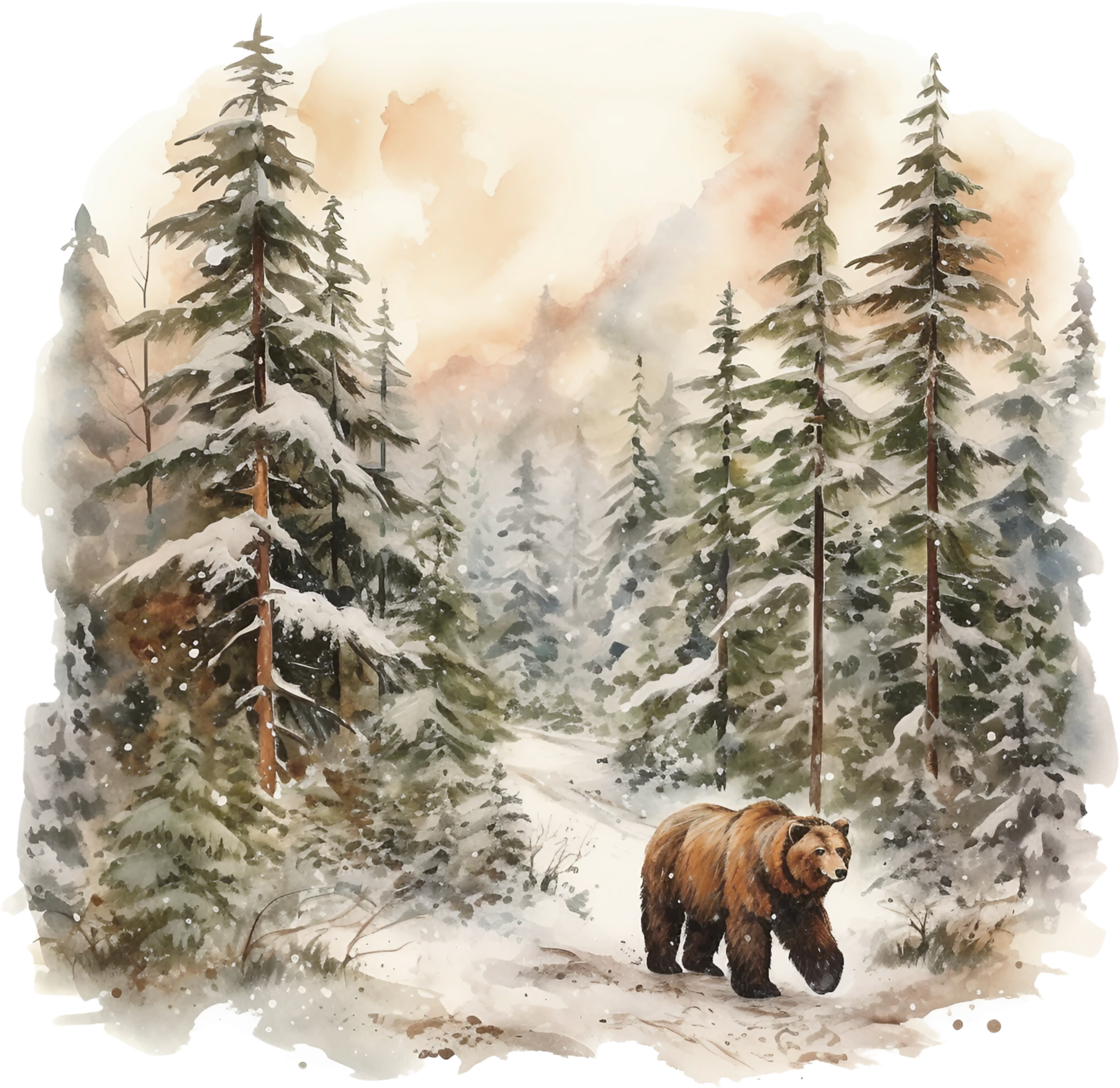The image is a striking winter scene depicted either as a painting or a digital art piece, featuring a brown bear walking along a snowy path in a forest. The tall pine trees, their branches heavy with snow, create a natural walkway, parting on either side to frame the bear. Set against a backdrop of fluffy white clouds tinged with orangey-pink hues, the wintry atmosphere is further enhanced by the snow-covered landscape and the contrasting colors of the bear's dark brown fur, the green trees, and the white and gray patches of snow. The bear, positioned towards the bottom right of the image, appears mid-step, with its left front paw raised, suggesting motion as it makes its way through this serene, snow-draped forest.